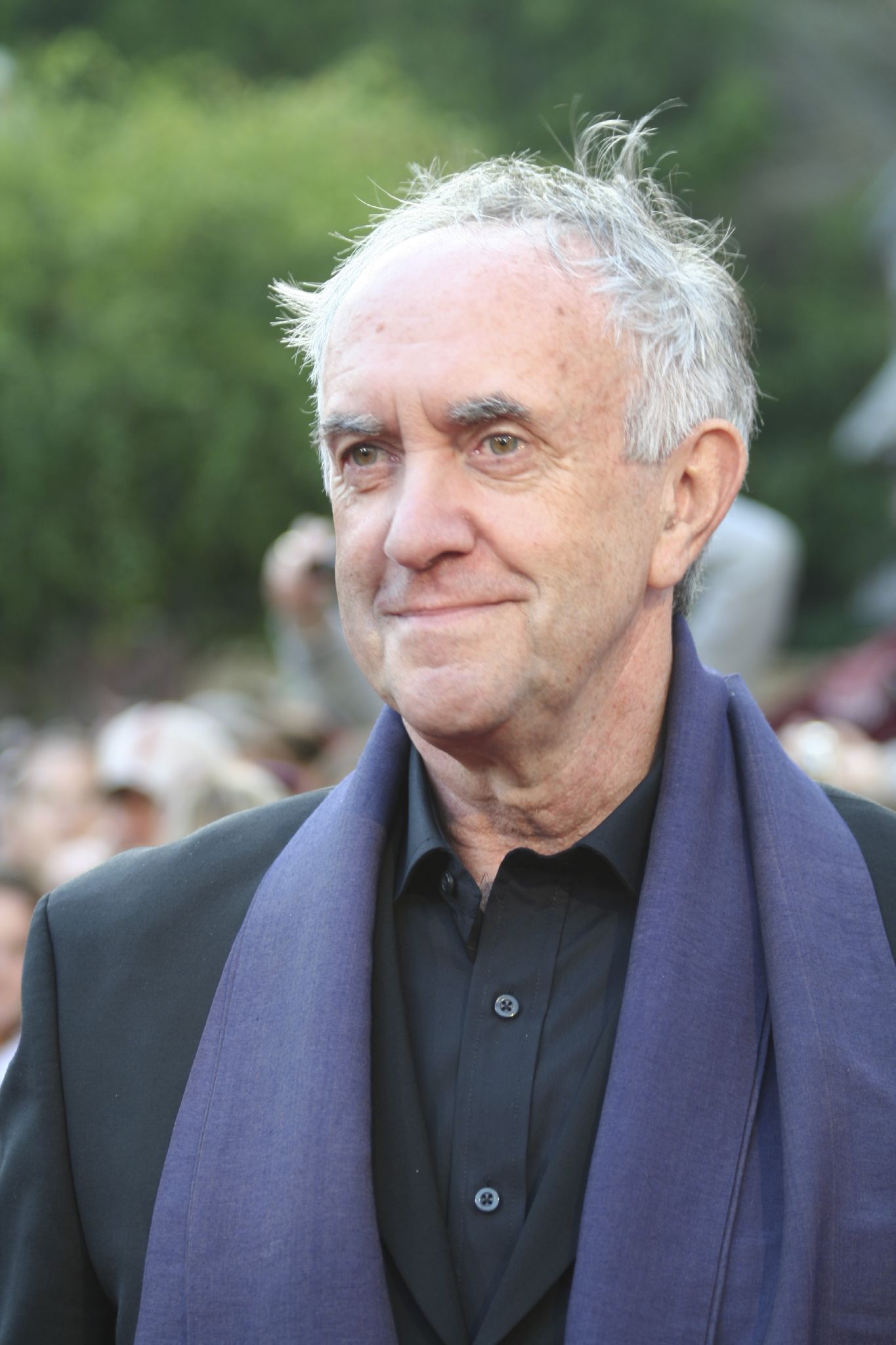This photograph captures an older white man with a receding hairline, displaying a mix of gray and black hair. His bushy eyebrows mirror this color blend. His long, wrinkled face with noticeable bags under his eyes is pointed slightly to the left, and he offers a closed-mouth smile. Dressed in a black button-down collared shirt and a dark suit jacket, he accessorizes with a navy blue scarf around his neck. Behind him, a crowd of people appears blurred, and above their heads, the bright green leaves of large trees are distinctly visible.